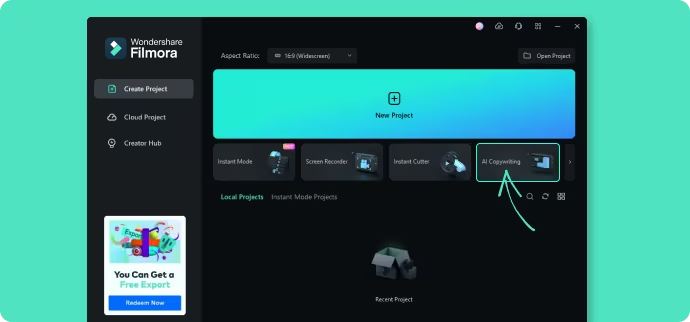Here is the detailed and cleaned-up caption:

---

The image features an interface with a predominantly blue background, displaying several UI elements and symbols. At the bottom section, a light blue highlight can be seen. 

In the top middle, white text reads "Expert Ratio 16:9 (Widescreen)." Below this, there is a large blue rectangle containing the text "New Project" with a plus symbol. To its right, options labeled "Instant Mode," "Screen Recorder," and "Instant Cutter" are listed. 

A blue arrow points towards the "Copywriting" feature nearby. In the top right corner, there is a circular icon next to a cloud symbol, possibly indicating a GitHub repository and a folder to open existing projects. 

At the bottom left, the text "Local Projects" and "Instant Mode Projects" is visible. Beneath this area is an icon of an open cardboard box, labeled "Recent Projects." A magnifying glass icon is present, along with scrolling arrows.

Towards the bottom, a light bulb symbol is visible next to the phrase "Create Pod Project." Scattered blue rectangles are interspersed throughout the background, giving the appearance of a dynamic interface. Additionally, colorful graphical elements depict a creative explosion effect. 

Finally, text at the very bottom mentions the availability of free team exports.

---